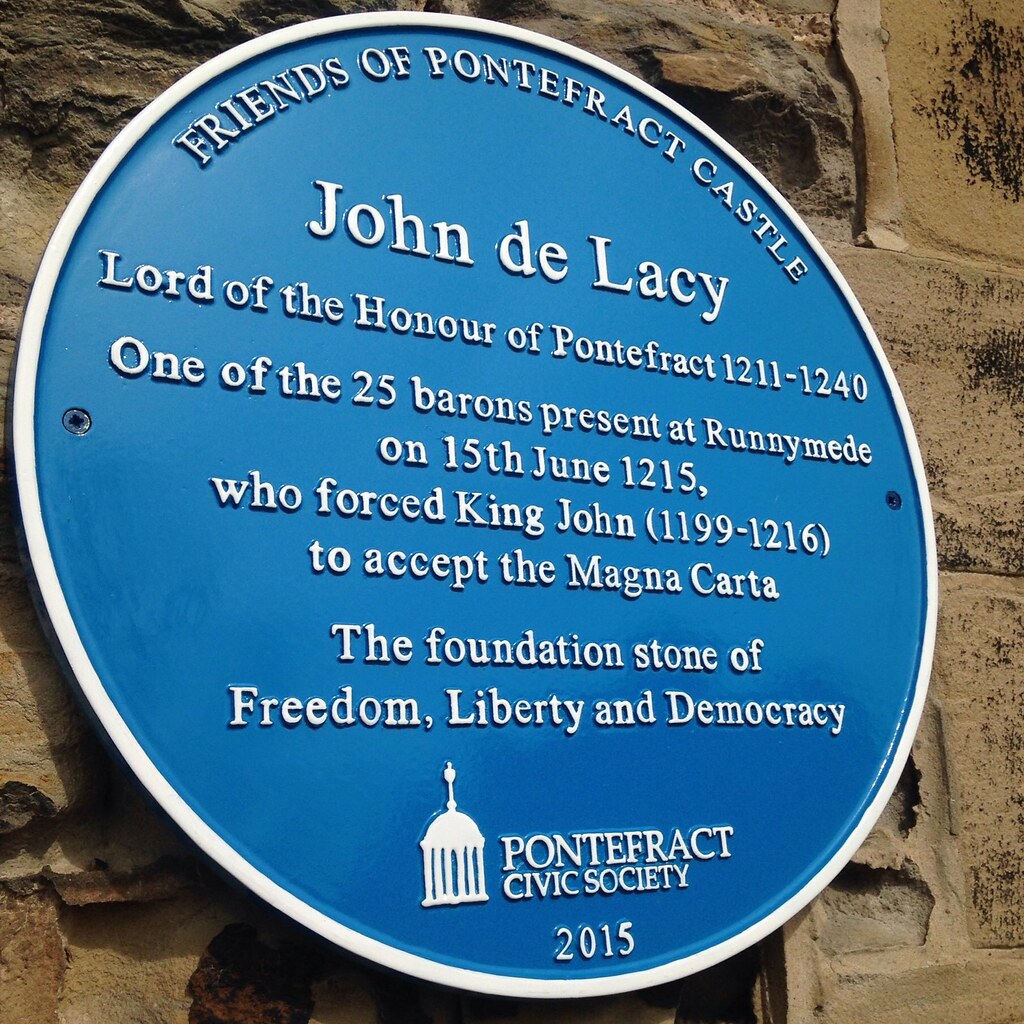The photograph captures a circular placard mounted on a rough, slightly chipped stone wall, secured by two large screws on either side. The plaque is dark blue with a white border and raised white lettering. At the top, the words "Friends of Pontefract Castle" are curved along the edge. Below, the inscription reads: "John DeLacy, Lord of the Honor of Pontefract 1211-1240, one of the 25 barons present at Runnymede on 15th June 1215, who forced King John (1199-1216) to accept the Magna Carta." The text continues: "the foundation stone of freedom, liberty, and democracy." At the bottom of the plaque, it reads "Pontefract Civic Society, 2015" and features a small emblem resembling the U.S. Capitol building with a figure at the top. There is a strong emphasis on the historical significance and contributions of John DeLacy and the foundational importance of the Magna Carta.